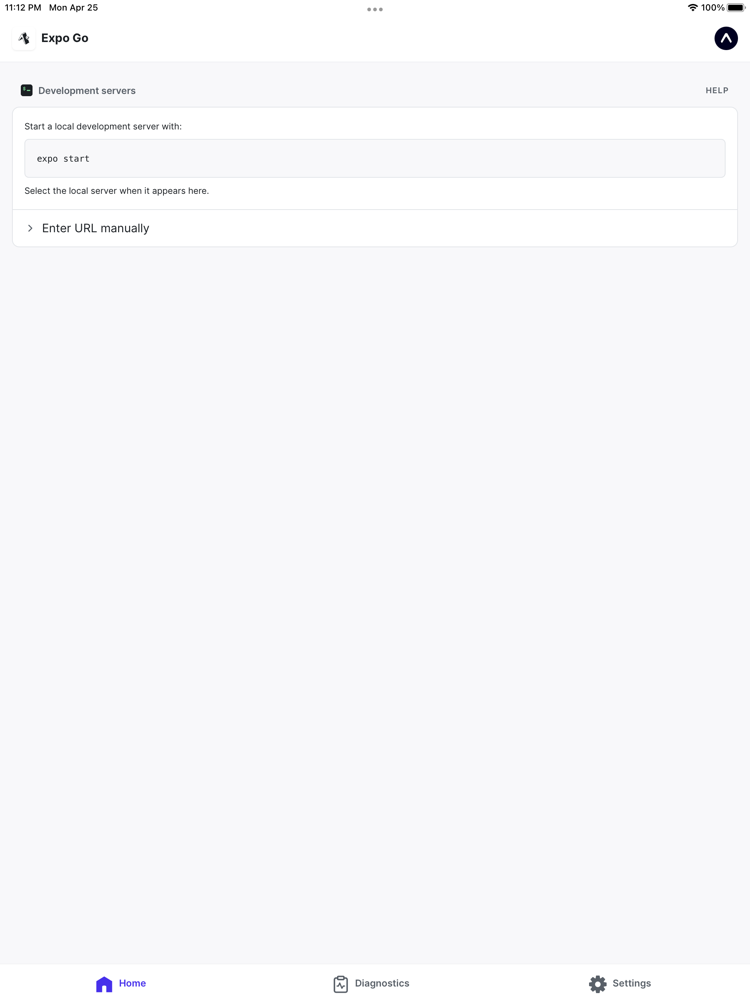The image showcases the Expo Go application interface on a mobile device, indicated by the presence of the status bar. The status bar at the top reveals the current time, 11:12 p.m., alongside the date, Monday, April 26th. The device is fully charged at 100%, with the service indicator and battery icon shown on the right side of the screen.

At the top center of the interface are three horizontal ellipses, likely representing a clickable menu icon. Below this, on the left side, the text "Expo Go" is displayed next to a small icon. On the right, a black circle with a white upward-pointing arrow is visible.

Further down, the section titled "Development Servers" includes the prompt: "Start a local development server with Expo Start. Select the local server when it appears here." Directly beneath this is an option labeled "Enter URL manually," accompanied by a left-pointing arrow.

The application's interface has a predominantly white or off-white background. At the bottom of the screen, there are three navigation buttons: a home button on the left with a house icon, a diagnostics button in the center featuring a clipboard with a graph, and a settings button on the right marked by a gear icon.

This detailed description provides a comprehensive look at the layout and functionality of the Expo Go application as displayed on the user's device.